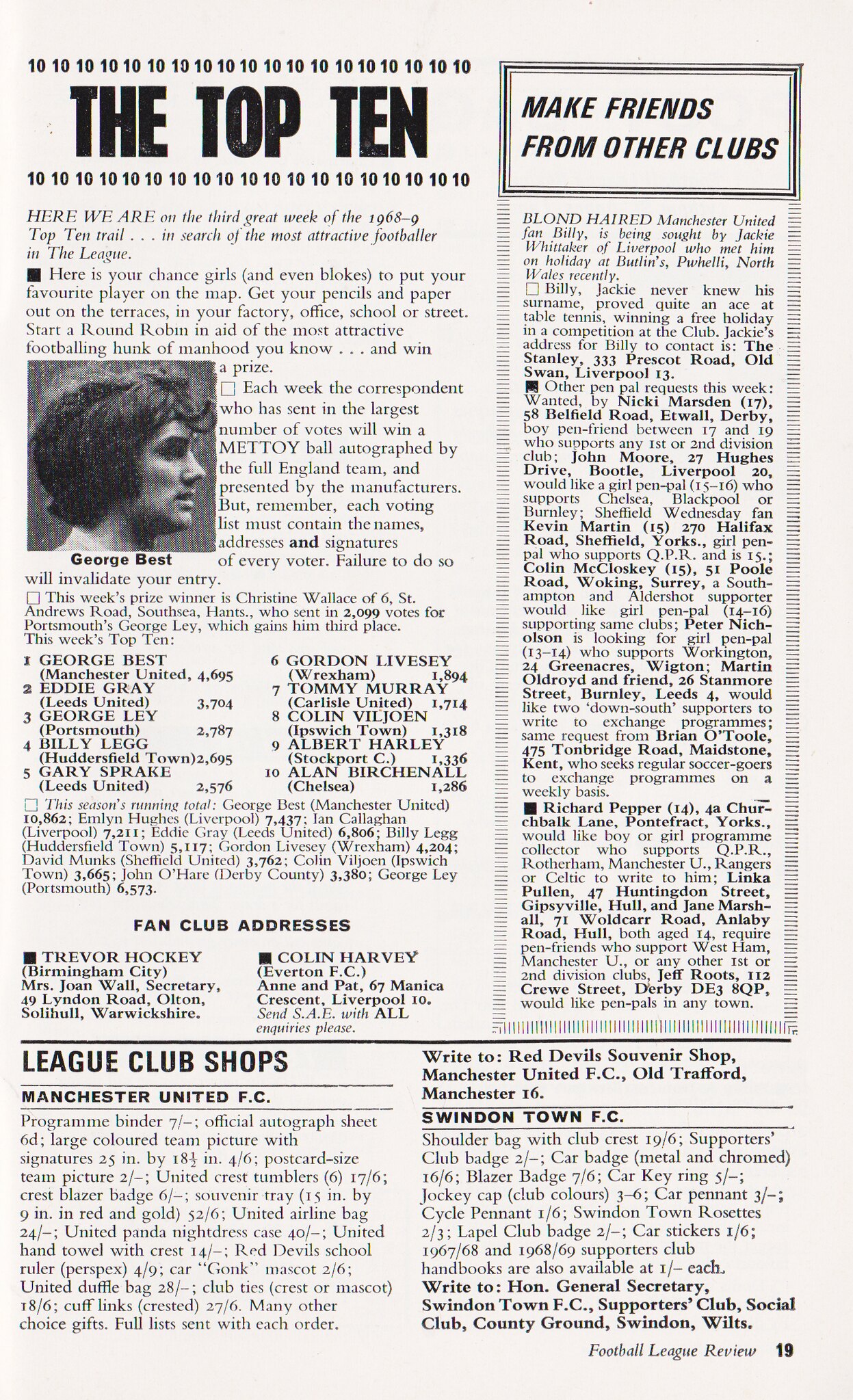The image is a cutout from a vintage magazine page, likely the "Football League Review," dating back to the third week of 1968. The off-white, cream-colored page features a bold, prominent headline, "The Top Ten," flanked by the repeated number '10' on the top and bottom borders. This headline kicks off a main article on the search for the most attractive footballer in the league, encouraging girls to vote for their favorite player by writing in from various locations like terraces, offices, and schools.

On the left side of the page lies a significant block of text and a monochrome photograph of George Best, a famous white footballer with mid-length hair, facing right. Underneath this article, there is a section for fan club addresses, notably mentioning Manchester United and Swindon Town, where fans can send letters.

To the right of the page, there's a black square headline stating, "Make Friends From Other Clubs," which introduces a pen pal program for football fans to connect with players like Trevor Hockey and Colin Harvey.

At the bottom of the page, there's a detailed section called "League Club Shops," listing items sold by Manchester United FC and Swindon Town FC, along with their prices. The bottom right corner of the page bears the words "Football League Review" along with the page number 19, solidifying its place within the magazine.